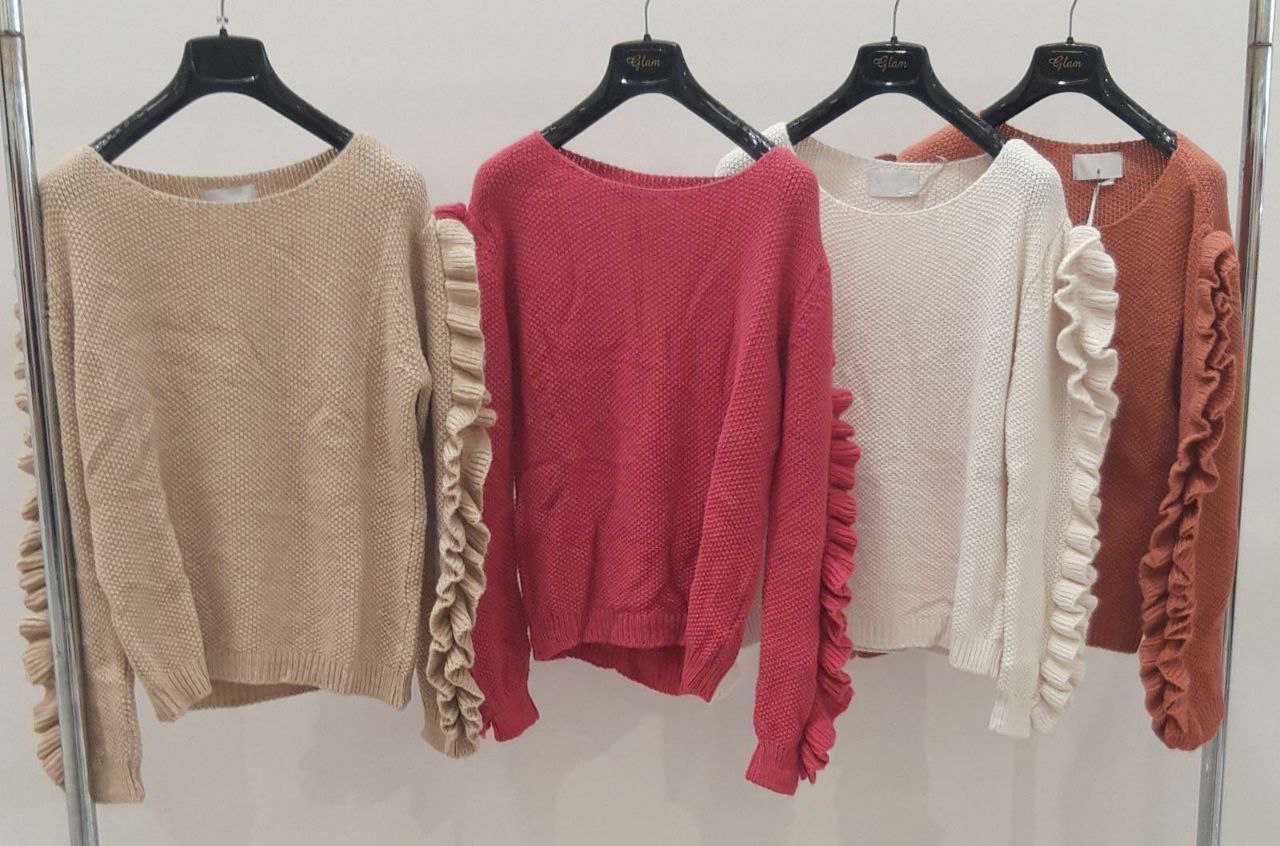The photograph features a metal clothing rack with four long-sleeve sweaters, each hanging on a black plastic hanger. The background is a white wall, allowing the sweaters to stand out prominently. Each sweater is of the same style and design, featuring a light textured fabric with ribbed bottoms and sleeves. Additionally, decorative ribbon-like fabric runs down the sides of both sleeves. The sweaters are arranged from left to right in the following colors: a light beige or tan, a dark pinkish red, a cream or white, and a dark brown, almost rust-like color. The hangers all bear the same logo, although it is not legible in the image. The sweaters are neatly aligned, providing a clear front view of each one.